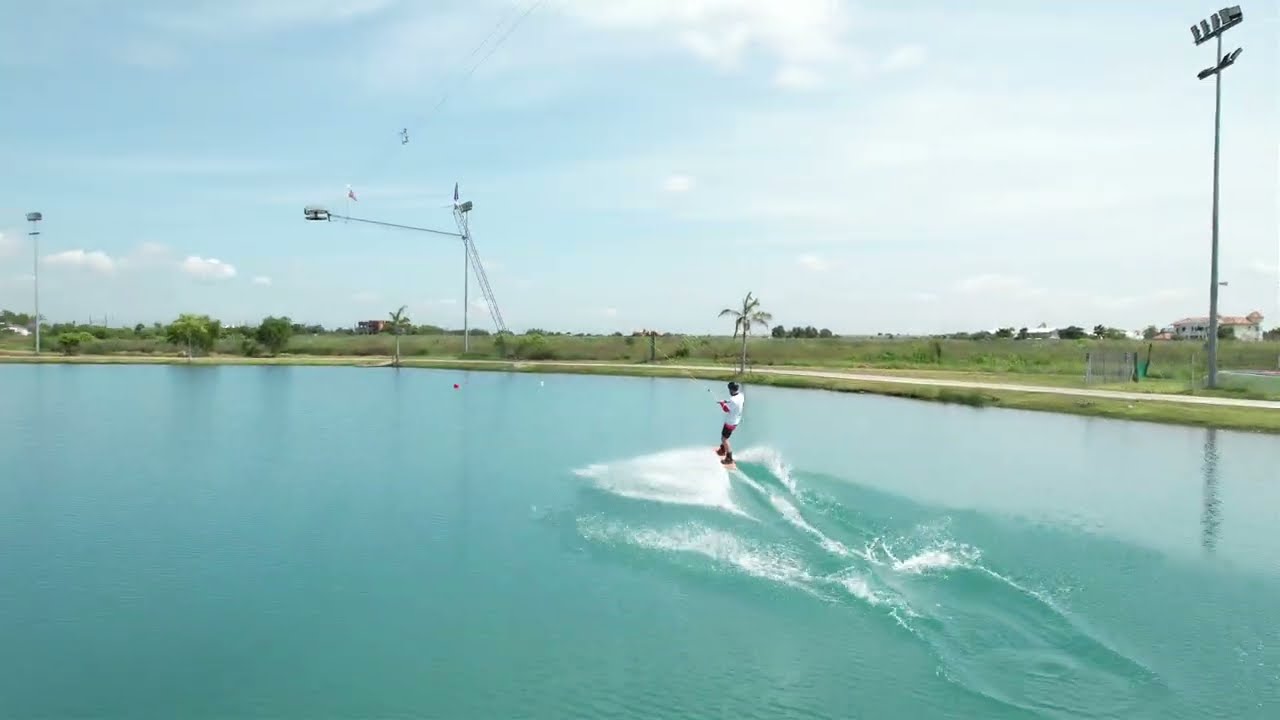The brightly lit, horizontally oriented photograph captures a summer day with partly cloudy blue skies above a large, clear body of light blue water. A person wearing a white t-shirt and black shorts is prominently featured in the middle of the water, engaged in wakeboarding or skiing. They are holding onto a long line attached to some structure, possibly a crane on a joist, creating a wake behind them as they ride a board across the water's surface. In the background, a lush green shoreline comes into view, dotted with low shrubbery, trees, and a pedestrian trail. The horizon line includes a couple of homes amidst the greenery and three lighting poles—one on the right, one toward the middle left, and another further to the left. There's also a lone palm tree in the distance. The image is vibrant, with a mix of blue, white, and green colors, providing a picturesque setting of a sunny, summer day.